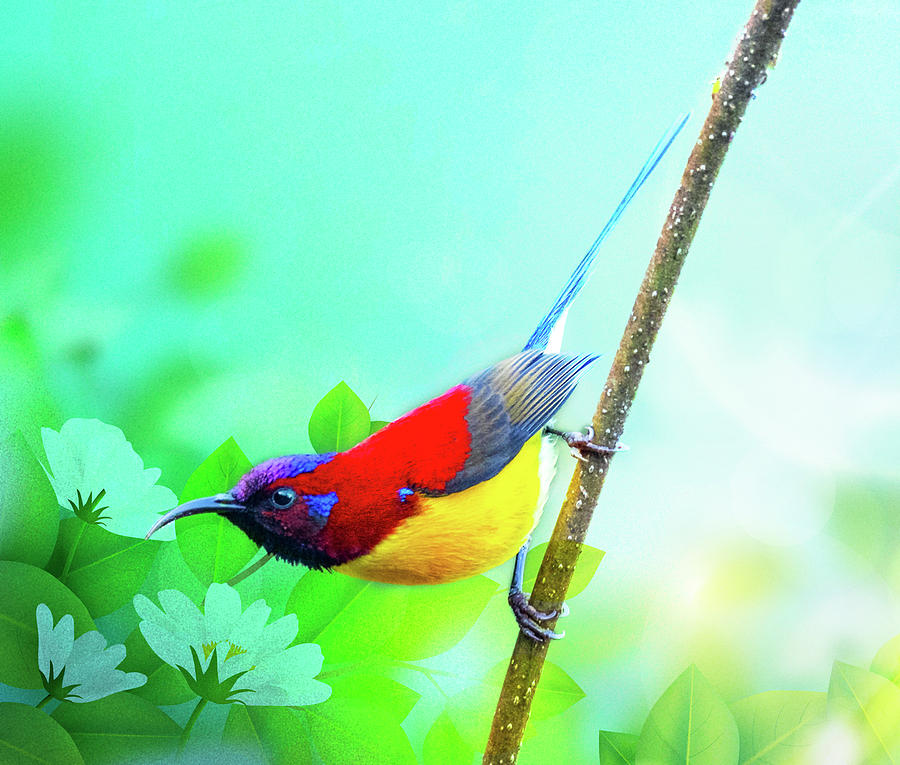This image features a stunning illustration that closely resembles a painted bunting. The bird is perched on a moderately sized branch, perfectly grasped by its blue feet, and leans over in a parallel posture to the base of the image. The bird's beak, a distinctive black curved into a subtle c-shape, points towards the left. Notably, the head transitions from a rich purple at the top to vivid blue around its eyes. The bird’s wings showcase a brilliant blend of red and blue tips, while its belly shines with a vibrant yellow. The tail is long and blue, adorned with intricate blue and yellow striations. The background offers an artistic blend of gradient shades between blue and green, dotted with detailed, white daisies with yellow centers surrounded by lush green leaves. The branch itself is brown with distinct white specks, enhancing the naturalistic setting. The finely detailed and possibly AI-generated nature of the image merges the boundaries of digital photography and high-quality digital art, encapsulating the delicate beauty of the painted bunting amid its serene surroundings.